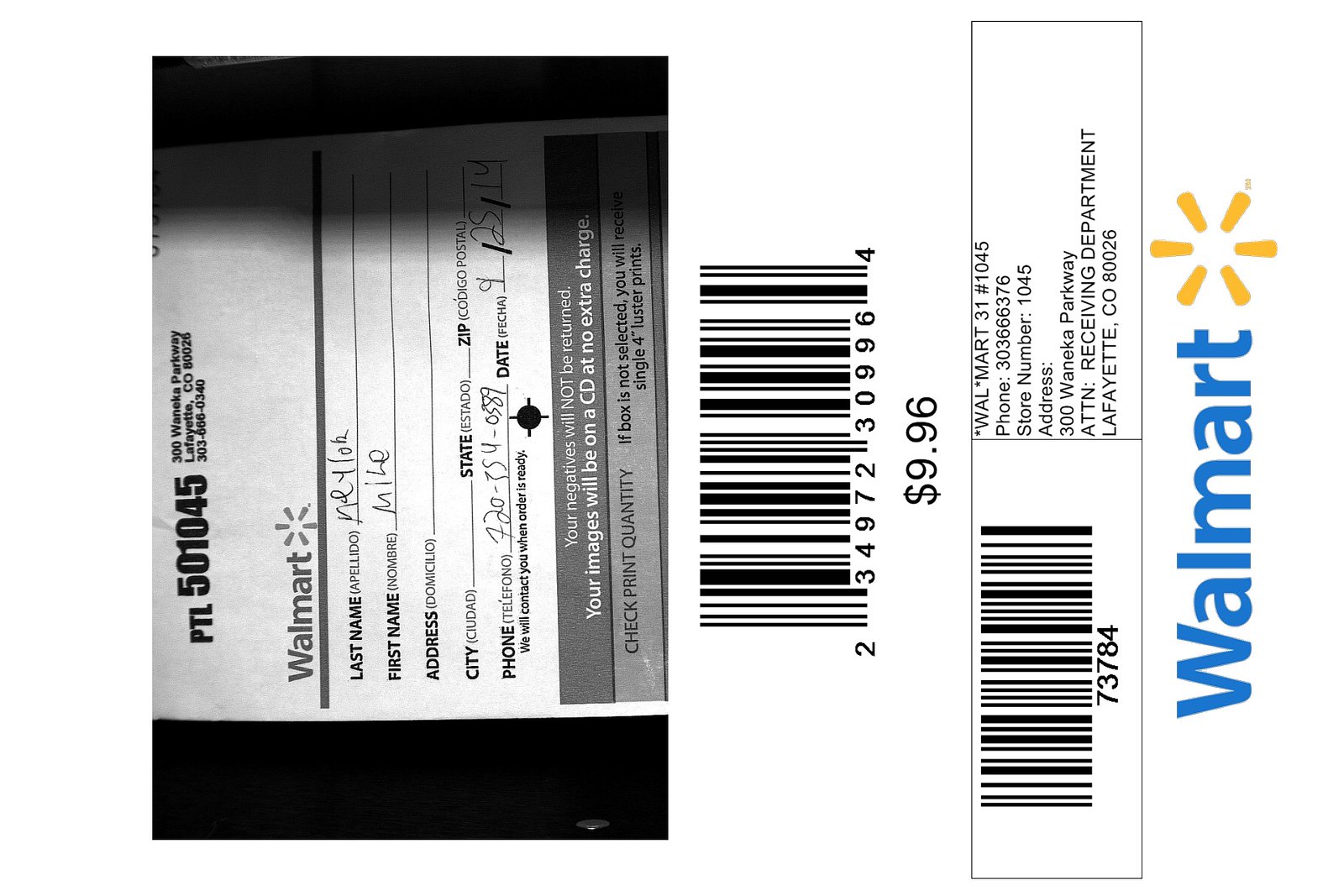The image displays a sideways photograph of a labeling sheet from a Walmart photo store order. The label comprises multiple sections, each providing detailed information about the order. The primary section of the label features the customer's name, "Natalo, Mike." However, key information such as the address and state is not filled in. A handwritten phone number, 720-354-0589, and the date, 9-25-14, are also present on this section.

Additionally, there are specific instructions indicating that negatives will not be returned and that images will be provided on a CD at no extra charge. It also mentions that if the print quantity box is not selected, the customer will receive a single 4-inch luster print. Adjacent to these details is a barcode labeled 234-972-309964, with a price of $9.96 noted alongside it.

To the right, there is a square containing another barcode, accompanied by text that includes "Wal-Mart 31, number 1045," and a phone number, 303-666-376. The store number, 1045, and its address at 300 Wanaka Parkway, Lafayette, Colorado, 80026, are also specified, directing attention to the receiving department.

The right-hand side of the sheet, oriented vertically, displays the Walmart logo in blue letters accompanied by the signature asterisk.